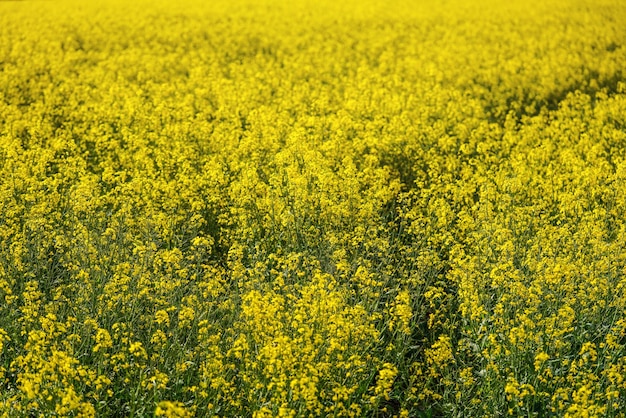This is a color photograph in landscape orientation, capturing a vast, sunlit field brimming with bright yellow flowers, possibly rapeseed or goldenrod. The scene is tightly packed from top to bottom and left to right with a continuous carpet of light yellow-gold flowers, blending into a concentrated blur of yellow in the distant horizon. In the foreground, thin green stems and leaves are visible, adding a touch of green under the dominant yellow. The view appears to be slightly downwards, as if taken from the center of the field, emphasizing the expanse and uniformity of the flowers. The photograph represents a realistic portrayal of this vibrant, lush field, bathed in sunlight.